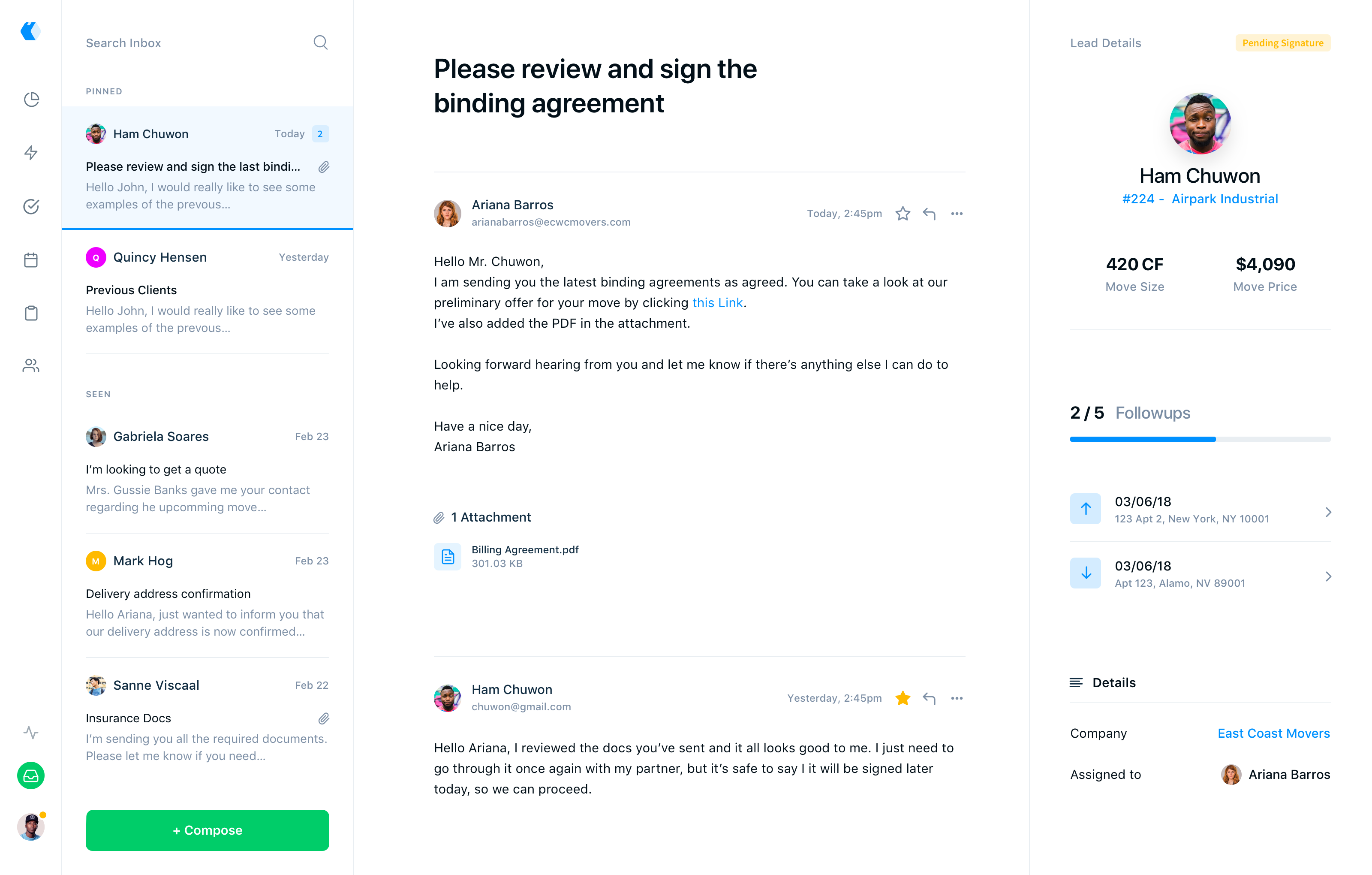In this screenshot, we observe a page from an email inbox featuring a detailed summary of a user's recent activity and correspondence. On the right-hand side of the image, the user's profile information is displayed prominently. The user is identified as Ham21, with an associated number 224, representing AIRPAC Industrial. Specific details of a transaction are outlined below: move size is indicated as 420 cubic feet, with a move price totaling $4,090. The follow-up action items show 2 out of 5 tasks completed. The relevant dates are listed as March 6th, 2018, with the location specified as 123 Apartments, New York, 10001.

The central portion of the image highlights an important message requesting action from the user: "Please review and sign the binding agreements." Additional messages in the inbox are visible, showing communication from and to various individuals, specifically Ham21, Quincy Henson, and Gabriela Stahls. This detail-rich snapshot captures essential aspects of a transaction process and user interactions within an industrial or corporate context.